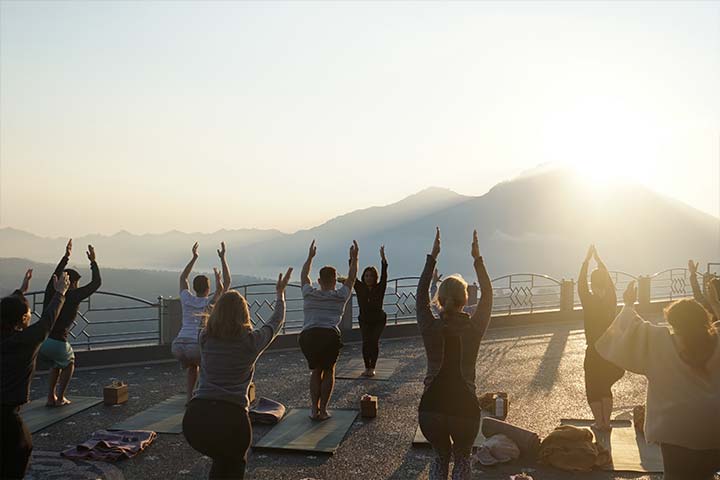The photograph captures a picturesque outdoor scene, likely taken shortly after sunrise, featuring a group of people engaged in a yoga session on a bridge or observation area. The participants, standing on rectangular yoga mats that cover a patterned ground, are arranged in rows with their arms extended upward and their knees slightly bent, facing away from the camera towards the sunrise. The yoga instructor, dressed in black, stands at the front, facing the camera and positioned in front of a fence that runs along the edge of the bridge, ensuring safety. Behind this fence, the image reveals a mountainous landscape, though the sun's intense glare in the upper right corner of the frame obscures much of the background detail, casting vibrant light and shadows. The sky above is clear, adding to the serene atmosphere of the early morning exercise. Scattered around the participants are various items like towels and small personal belongings, adding a touch of casual realism to the scene.